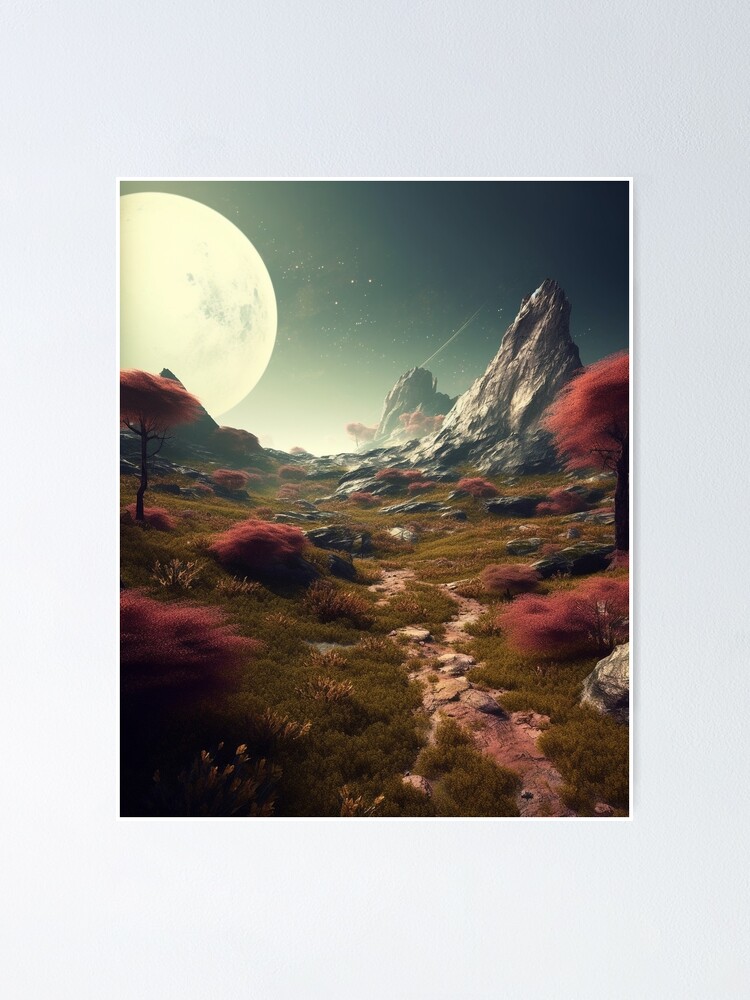The image is a detailed and captivating digital artwork likely depicting a fantastical, faraway world under a dark, starlit sky. Dominating the top left is an enormous, exaggeratedly large moon, its bright white surface dotted with darker craters, which casts an ethereal glow across the entire scene. The night sky is adorned with numerous stars and the faint trail of a shooting star, adding to the otherworldly atmosphere.

Beneath the moon, the landscape slopes downward, featuring dramatic cliffs in varying shades of gray. These cliffs transition into a plains-like area covered in short grass and mossy patches. Bright red bushes and trees provide a striking contrast to the predominantly gray and green landscape. The trees, with their vivid red foliage, extend into the distance, eventually merging with rock formations.

A subtle stream winds its way through the terrain, parting the green land and weaving around scattered, large gray rocks. This rocky plain is illuminated by the radiant moonlight, which highlights the texture and details of both the rocks and the vibrant plant life, creating a surreal and enchanting tableau.